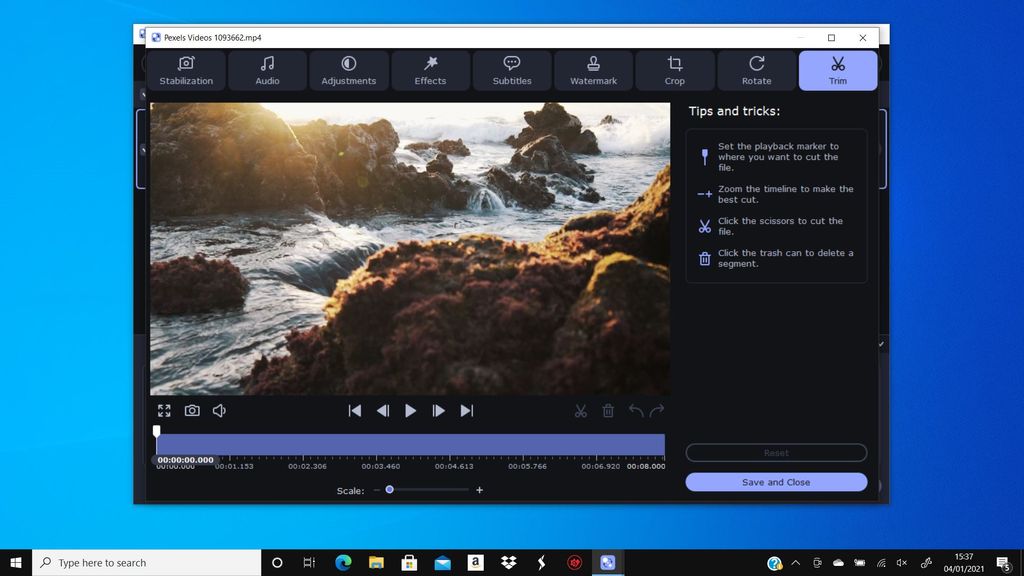The image displays a video editing interface set against a vibrant blue background. The main video window, currently minimized, features a serene yet rugged seashore scene, capturing waves rhythmically crashing and receding. The video appears to be a personal or user-generated clip from a platform like "pixel videos," indicated by the screen's title.

At the top of the interface, a toolbar offers various editing options, including "Stabilization," "Audio Adjustments," "Effects," "Subtitles," "Watermark," "Crop and Rotate," and "Trim." The "Trim" function is active, as highlighted by the interface.

Beneath the main video window, playback controls like "Play," "Fast Forward," and a blue progress tracker display the current timestamp of the video. To the right, a "Tips and Tricks" section provides guidance on using the trim feature: it advises setting the playback marker to the desired cut point, zooming in on the timeline for precision, and using the scissors icon to cut or the trash can icon to delete a segment.